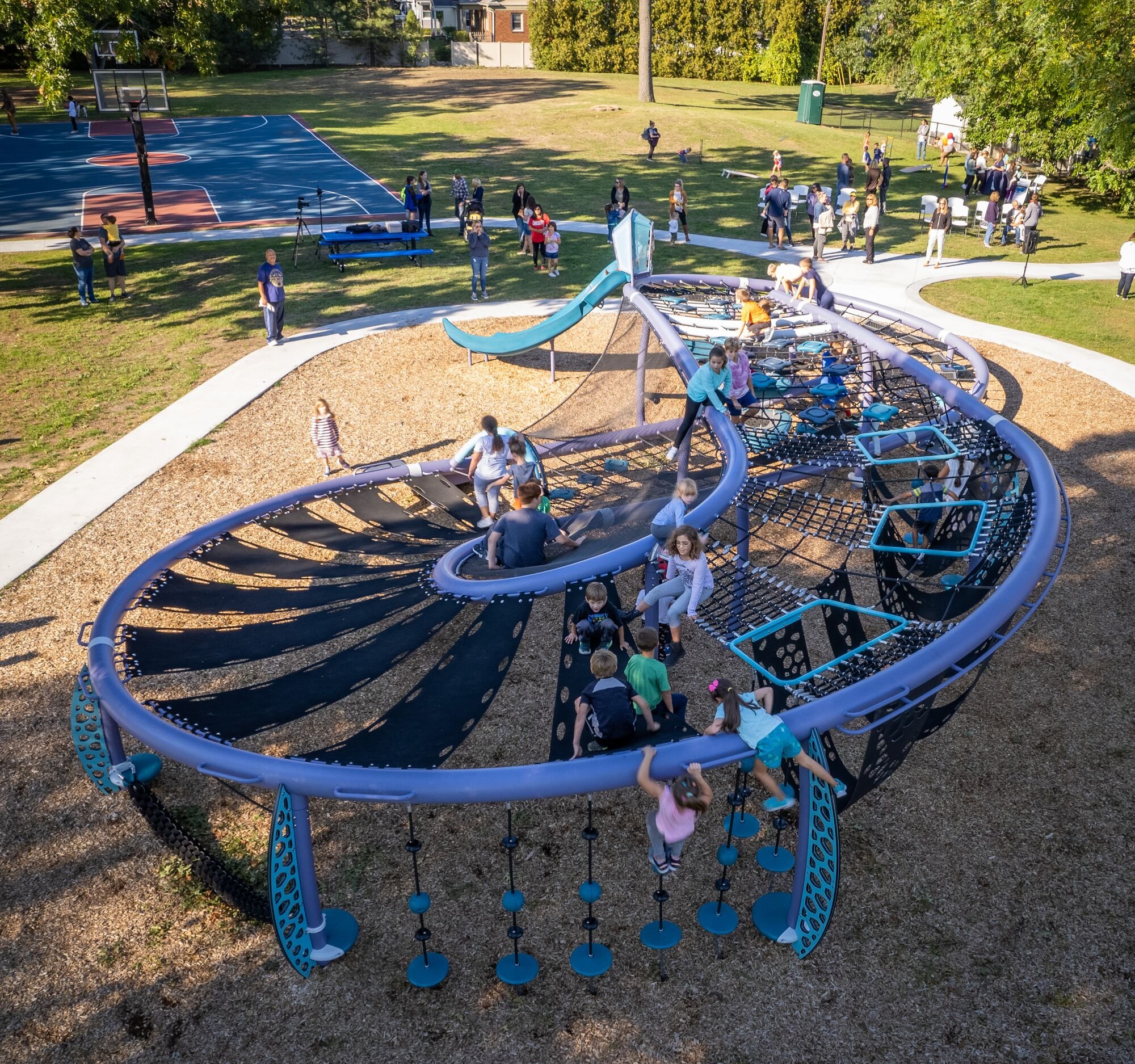This outdoor photograph captures a lively playground from an elevated perspective, providing a comprehensive view of the various elements within the scene. In the foreground, a prominent blue jungle gym structure dominates the image. This intricate play structure starts from the center and curves to the left before looping back to the right, featuring numerous nets and black tarp-like bridges designed for children to crawl across. Several children are visible on these nets and bridges, actively engaging with the equipment.

The playground surface consists of a brown sandy or dirt area that cushions falls, with cement walkways curving along the perimeter to the left and leading off into the distance on the right. Surrounding the playground, there's an expanse of green grass dotted with numerous trees and lampposts. Scattered adults stand to the left and right of the playground, observing or waiting.

In the upper left of the image, a blue basketball court with two hoops is clearly visible, while the top right portion showcases more trees. Towards the center top of the photograph, a building can be seen in the background, flanked by additional greenery and shrubberies. This detailed, bustling scene captures the vibrant energy of children at play and the supporting environment around them.